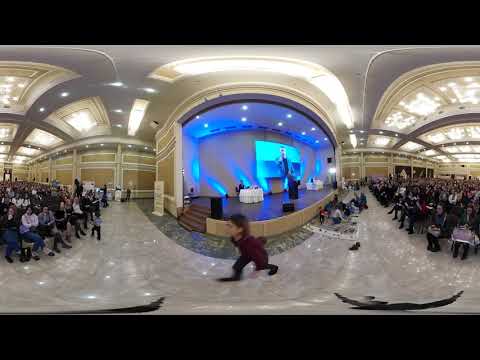This color fisheye photograph, likely taken from a monitor or security camera, depicts a large conference hall with a warped, distorted view across three stitched images. The scene is centered on a stage dominated by recessed and canned lighting that creates significant glare and reflections against the beige and gray ceiling. The stage is highlighted with blue lighting, adding a dynamic visual element. In the center rear of the stage, there is a small table covered with white sheets, flanked by a dark podium. A person dressed in a maroon shirt and black pants is captured mid-stride at the right bottom center, walking towards the left. The lower black horizontal strip and rounded angle suggest a fisheye lens or associated filter is applied. The audience, dressed in professional attire, occupies rows of chairs on both sides, attentively observing the proceedings. The hall's gray carpeting and ceiling lighting are clearly visible, setting an atmosphere typical for a conference or a performance event.